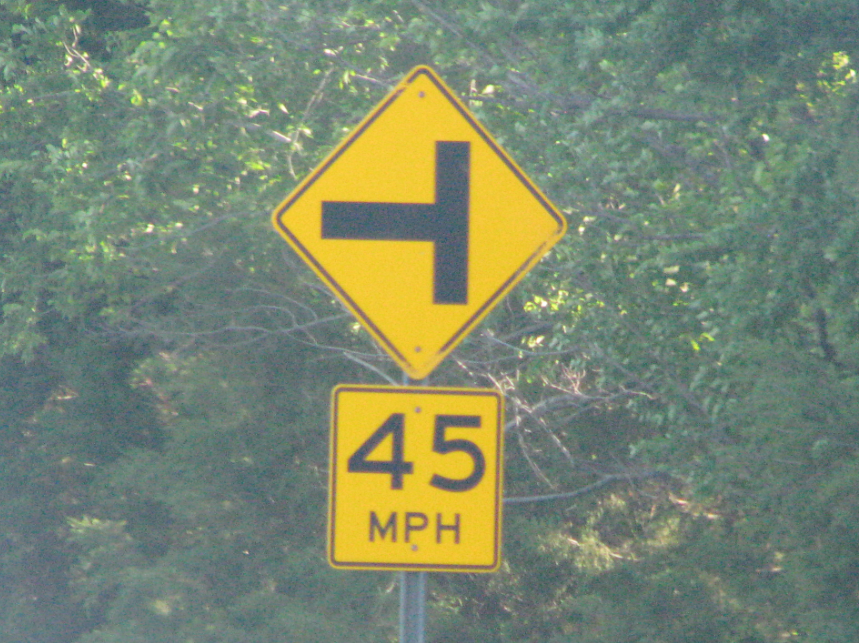This photograph captures a standard road sign positioned on the side of a road, supported by a gray metal pole. The sign consists of two distinct components. The upper segment is diamond-shaped with a yellow background and a thin black border, indicating an upcoming T intersection. The black symbol on this segment shows the T turned 90 degrees to its side, with the top part oriented vertically to the pole. Below this, there is a rectangular sign with the same yellow background and black border. It prominently displays the number "45" in large font, while "MPH" in smaller font underneath indicates the speed limit in miles per hour. The backdrop of the image comprises dense foliage with trees, branches, and thick brush, adding a natural setting to the scene.